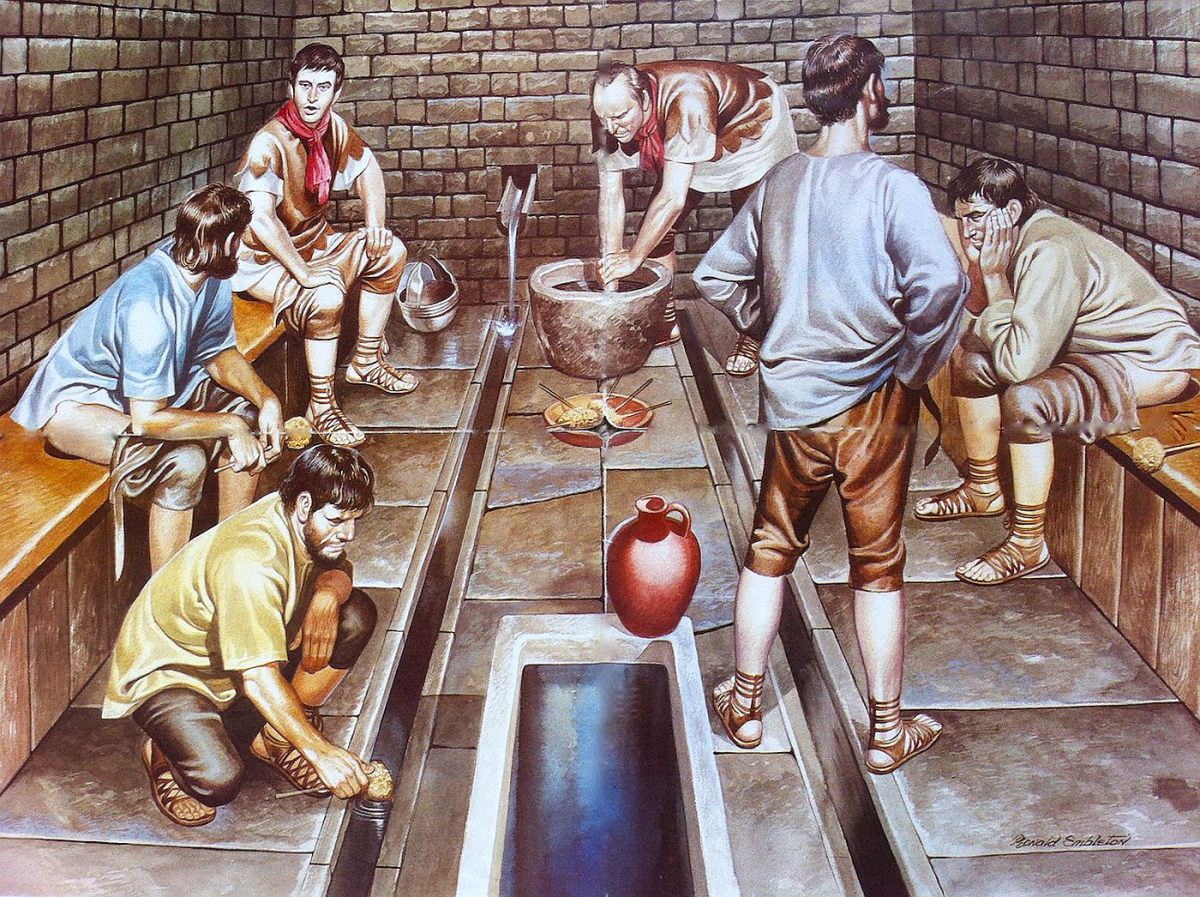The painting portrays an ancient Roman latrine scene, where six men, clad in tunics with culotte shorts and lace-up gladiator sandals, engage in various activities. Set within a stone-walled room, the image features wooden benches on both sides, with three men seated on each. Two men on the left converse, while a man on the far right sits facing away. Central to the scene is a giant stone basin, into which a man scrubs, perhaps washing himself or an object. Another man crouched at the front appears to be operating a nozzle or spout. Water pours from trenches that run across the floor, emphasizing the room's utilitarian purpose. Notable details include red handkerchiefs worn by two men and a helmet resting on the ground, suggesting a sense of uniformity or teamwork among them. The precise rendering of the men's attire and the detailed interior elements evoke a vivid sense of daily life in ancient Rome.